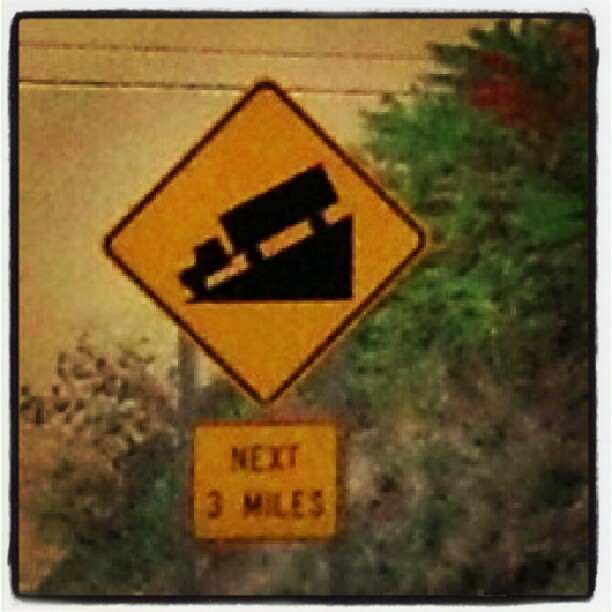The image depicts a somewhat blurry, low-resolution outdoor photo of a warning street sign against a natural backdrop, cautioning semi-trucks about a descending roadway stretch ahead. The focal point is a diamond-shaped, yellow sign with a black outline, illustrating a truck descending a steep slope, indicating a potential runaway truck hazard. Below the diamond sign, another yellow sign contains the black text "Next 3 Miles," also bordered in black, cautioning about the length of the descent. Both of these signs are mounted on two metal poles. In the background, a mix of green and brown hillside with some bushes and trees is visible, complemented by telephone or power lines crossing the image horizontally at the top. The entire scene appears framed as if taken with an instant film camera, adding a vintage grainy texture to the image.